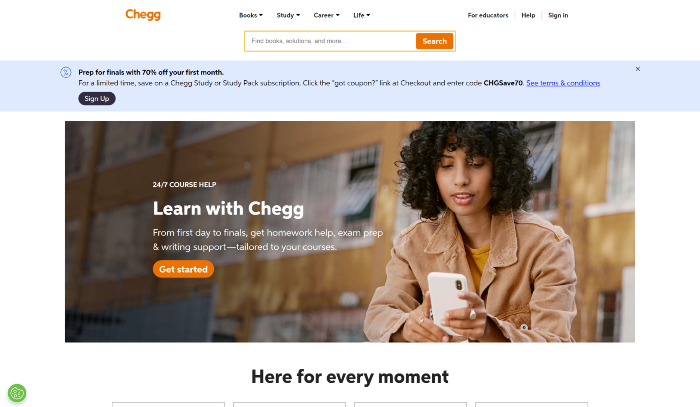Here is a revised and detailed caption for the described image:

---

This image is a cropped screenshot of the Chegg desktop webpage. Dominating the top of the page is the Chegg logo in vivid orange letters. Centered beneath the logo are four primary categories: Books, Study, Career, and Life, each accompanied by a drop-down menu for further navigation.

Just below these categories, there is a prominently placed search bar. The search bar is outlined in orange and features a matching orange search button situated on its right side.

Towards the top right corner, there are three key options labeled "For Characters," "Help," and "Sign In." There is also another variation where these categories are labeled "For Educators," "Help," and "Sign In."

Directly underneath the header section, there is a large blue promotional box. This box includes a small X icon in its top right corner, presumably for closing the ad. On the top left of this blue box, there is a blue icon, and to its right, a bold black message reads, "Prep for Finals with 70% off your first month."

Further down within this box, the text mentions: "For a limited time, save on a Chegg Study or Study Pack subscription. Click the Get Coupon link at checkout, and enter the code," with the applicable code highlighted in bold text. Additionally, there is a "See Terms and Conditions" hyperlink in blue.

Below this promotional message, there is a blue sign-up bar inviting users to take action.

The body of the webpage features a large, visually captivating photo backdrop. The backdrop displays a woman engrossed in her phone, standing in front of an academic building, which gives the impression of a college or university setting. On the left side of this backdrop, text reads "24-7 Course Help, Learn with Chegg," followed by an orange "Get Started" button located towards the bottom left.

---

This detailed caption clearly describes the visual elements and layout of the Chegg webpage, ensuring a comprehensive understanding for the reader.